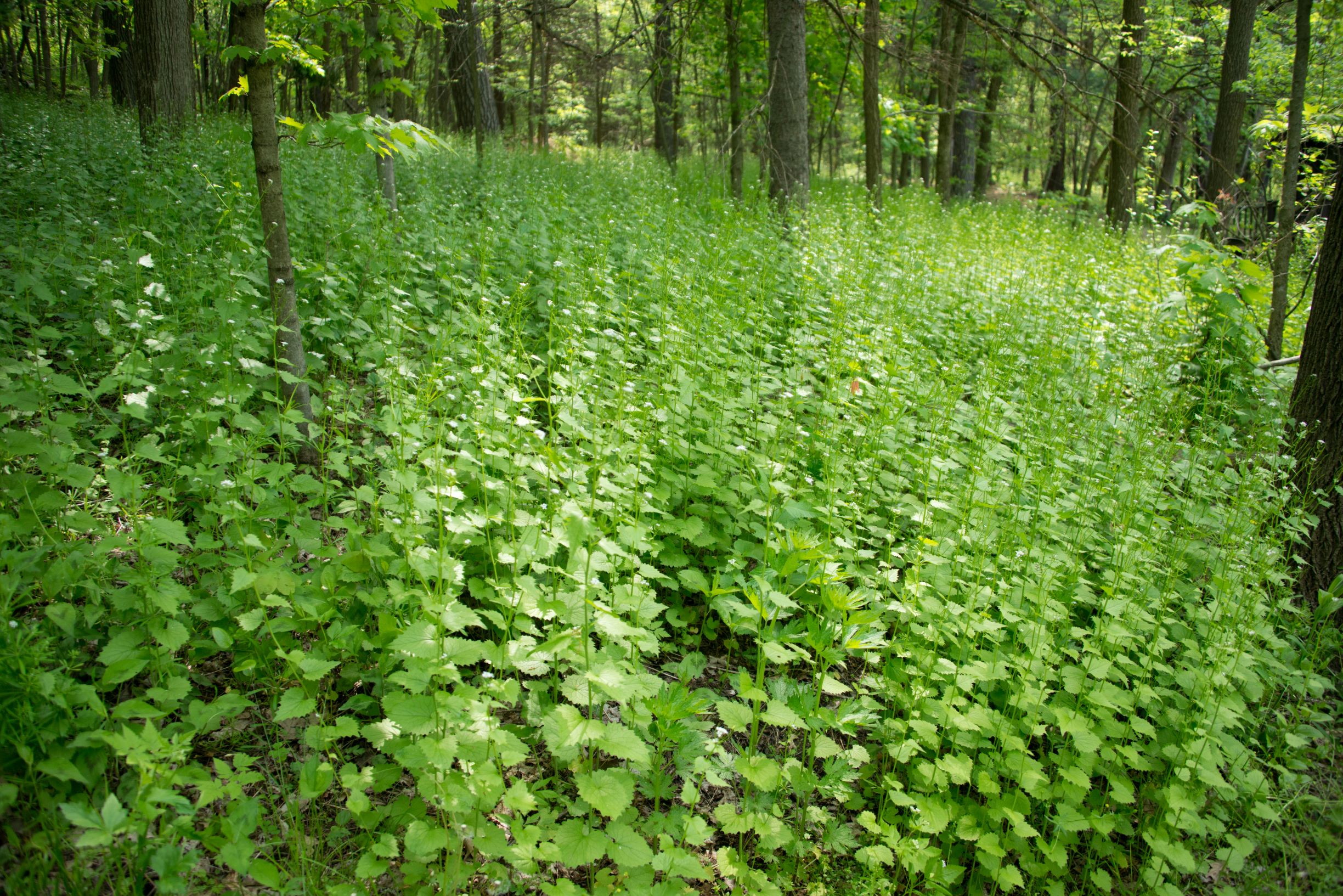This landscape-oriented photograph captures a vibrant wooded area bathed in daylight. The scene is predominantly dominated by a lush, green forest floor uniformly covered with tall, leafy plants. These plants, reaching about a couple of feet high, have serrated teardrop-shaped leaves that create a dense, almost carpet-like appearance across the entire slightly inclined hillside. Interspersed among these verdant plants are several skinny trees with thin trunks, providing a vertical contrast to the lush greenery below. Notably, the left side of the image features white leaves and small flowers, while the background hints at yellow leaves mingling among the tree foliage. The overall visual is a rich tapestry of green hues with occasional splashes of white and yellow, encapsulating a serene, natural forest environment.